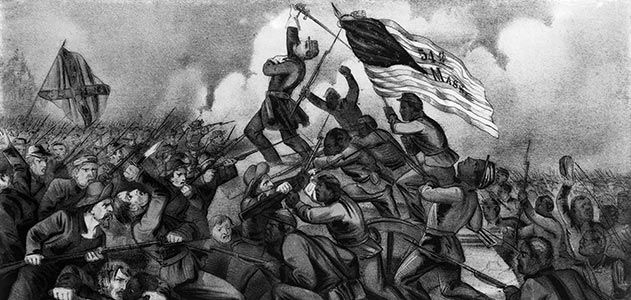This black-and-white artwork vividly illustrates a chaotic Civil War battle. The scene is dense with a mass of men engaged in fierce struggle, filling the frame. On the left-hand side, soldiers wearing military uniforms are prominently holding up a Confederate flag, marked with a dark black X against a lighter background. The confusion of war is evident, with smoke and billowing clouds dominating the backdrop, creating a gray and white haze that envelops the entire setting.

In the center, another flag stands out amid the turmoil—this one resembling the American flag, though it bears the numbers "544" and partially legible text starting with an "M," suggesting it might label a specific regiment. The flag bearer, caught mid-motion, appears to be trampling over other figures, emphasizing the chaos. Nearby, a man, likely an officer given his distinguished uniform and white gloves, is visibly wounded, clutching his chest as a sword slips from his grasp, capturing the moment of his fall.

The right-hand side of the image is a swarming sea of varied individuals—some in civilian clothes, adding to the sense of disorder and packed intensity. Amidst this, expressions of anger and desperation are etched onto the faces of the combatants. The right side appears to be rushing towards the left, likely indicating a charge or retreat. Overall, the image powerfully conveys the brutal and frantic nature of Civil War combat, the palpable tension of conflict, and the human emotions caught in its wake.